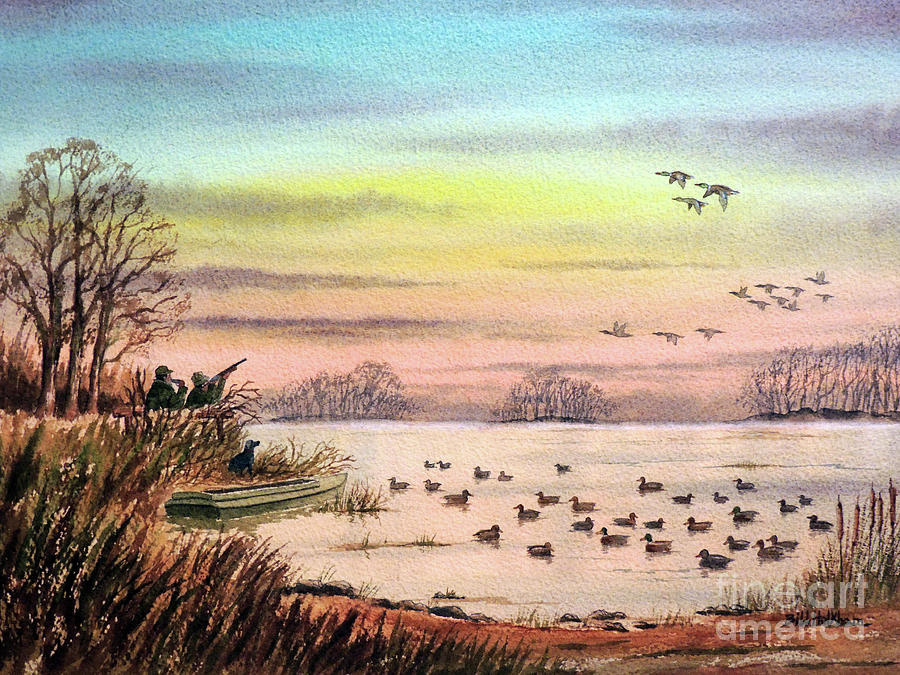This horizontal rectangular painting, labeled "Fine Art America" in white text at the bottom right corner, vividly captures an outdoor hunting scene. The composition features a serene river with numerous ducks swimming on its surface. The painting's foreground showcases a brown, dirt-covered shore, some patches of weeds, and a raised area on the left side with a hunting blind. Two hunters dressed in green jackets and hats occupy the blind, with one man blowing a duck call and the other aiming his shotgun at a flock of ducks flying through the sky. Nearby, a boat rests alongside the shore, with a dog poised at the water's edge, attentively watching the ducks. The background reveals a sweeping, picturesque marsh landscape adorned with an array of trees. The sky above transitions from a purple-gray clouded top to shades of blue, yellow, and pink, contributing to the overall tranquility and perfection of this art piece.